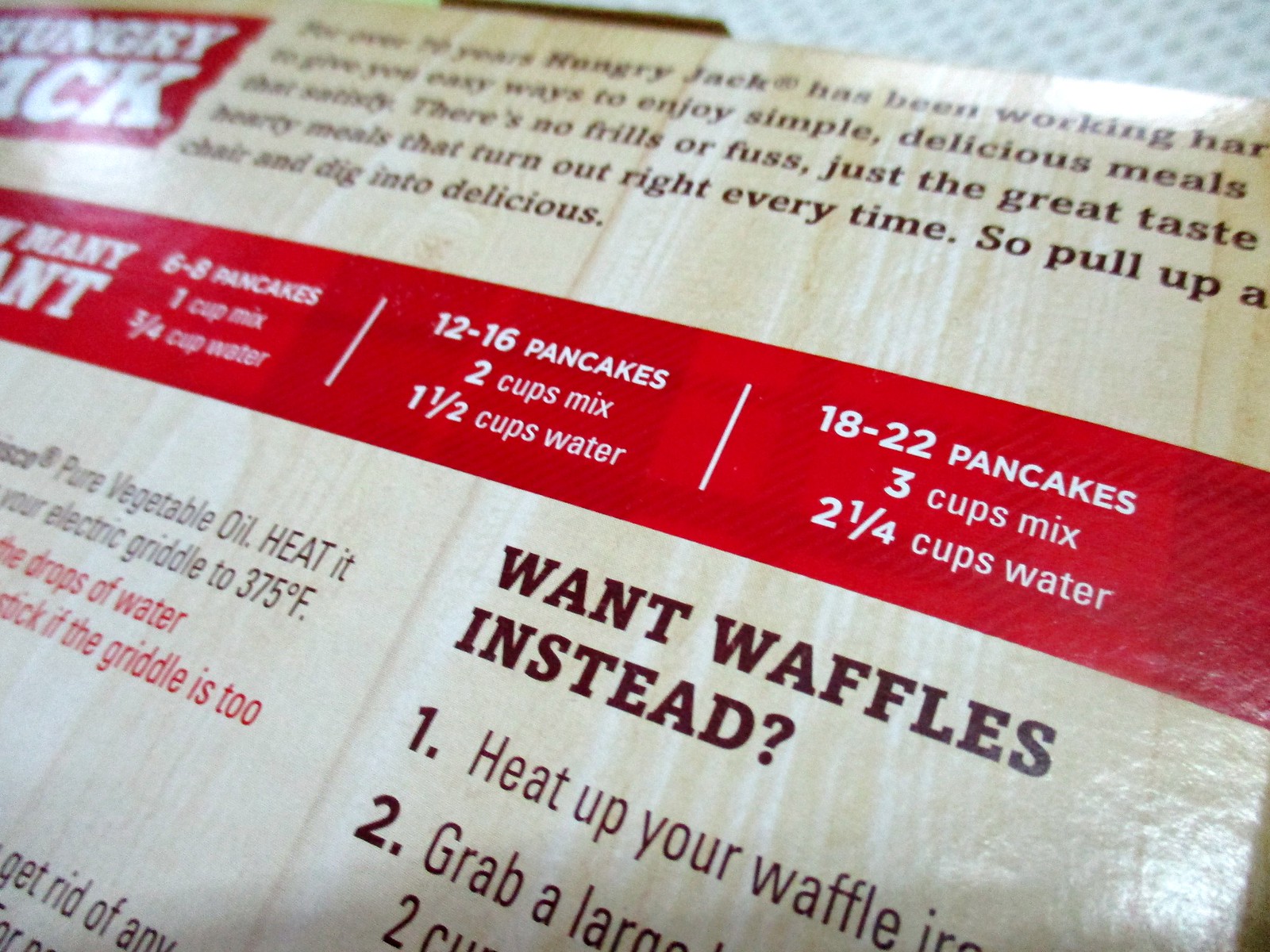The image is a close-up photograph of the back of a Hungry Jack pancake mix box, taken at an angle that cuts off some of the text and blurs certain details. In the top left corner, the Hungry Jack logo is visible, partially captured in a red rectangle with "Hungry" in one line and "Jack" in the next. At the very top of the box, there's black text that starts with "For over 10 years, Hungry Jack has been working hard" to make sure breakfast is simple and satisfying. Below this, the middle of the box features a detailed section about different sizes and quantities of pancake servings: "six to eight pancakes, one cup mix, three-fourths cup water," "twelve to sixteen pancakes, two cups mix, one and a half cups water," and "eighteen to twenty-two pancakes, three cups mix, two and a quarter cups water." Underneath, further instructions get truncated, mentioning "pure vegetable oil," an "electric griddle to 375°F," and something about "water drops." Towards the bottom, a clear but partial instruction reads, "Want waffles instead?" followed by "heat up your waffle" before the text is cut off.